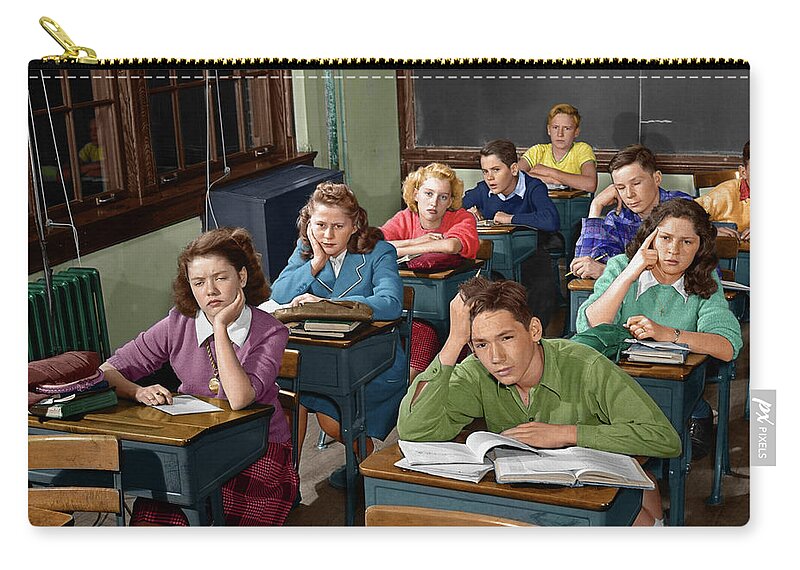This image is a detailed depiction of a vintage classroom scene printed on a coin purse with a golden zipper at the top, complemented by white stitching. The classroom, viewed from the teacher's perspective at the front, features about ten school children dressed in attire reminiscent of the 70s or 80s, with long-sleeved outfits and sweaters. They are seated in two rows at dark gray metal desks with wooden tops. Many students appear bored and confused, resting their heads on their hands or staring off into the distance. At the back of the classroom is a black chalkboard, while to the left are two wooden-framed windows and a green radiator in the bottom left-hand corner. A label in the right-hand corner of the bag bears the "PX" symbol and the text "pixels" in white against a gray tab. The scene captures a moment of mundane classroom life, enhanced by the nostalgic and somewhat melancholic expressions of the students.